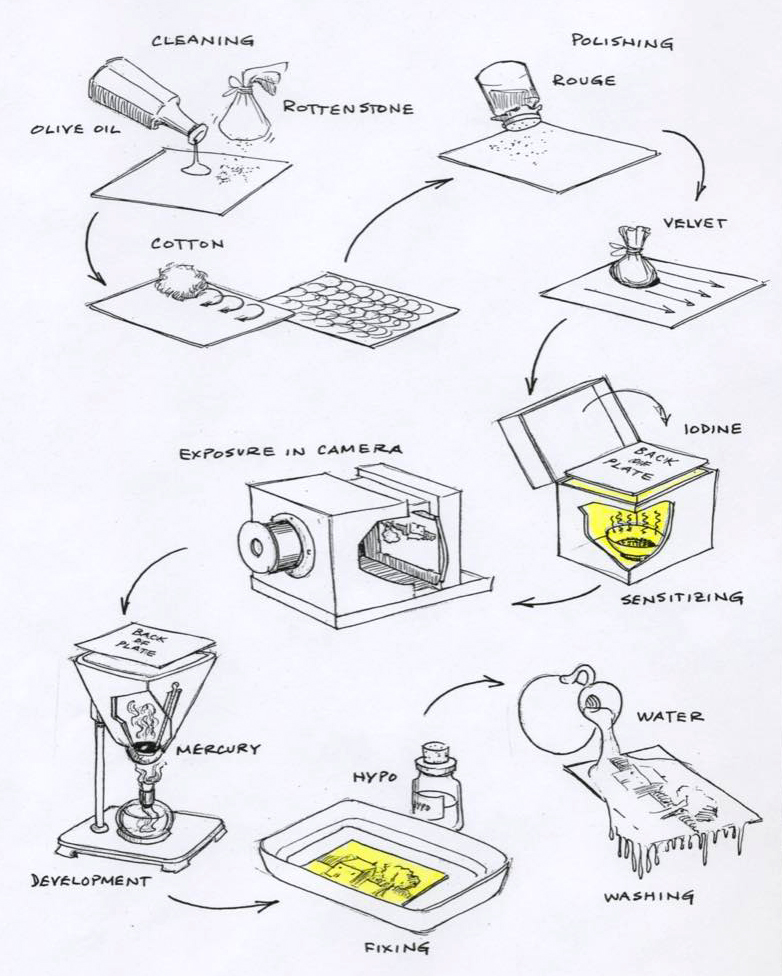The drawing depicts a detailed, traditional hand-drawn infographic for developing photographs using historical techniques. Moving in a clockwise direction and forming a backward S shape, the diagram illustrates each step of the process. At the top, a bottle of olive oil pours onto a surface labeled "rotten stone," represented by a pouch. An arrow points to a cotton ball, used to clean the surface in circular motions. This leads to polishing with rouge, followed by smoothing with a velvet sachet. The plate is then placed in a box of iodine for sensitizing—illustrated by rays emanating from a bowl inside the box. 

Subsequently, the sensitized plate is placed into a camera for exposure. The developed plate is then transferred to a container where mercury development occurs, shown with a flask and the plate situated above it. Following the development, the plate is immersed in a solution labeled "hypo" for fixing, depicted as soaking in a large tray. Finally, the plate undergoes a water wash to complete the process. The entire image is rendered in black and white with a pale blue background, and features selective yellow highlights in the iodine sensitizing and hypo fixing sections.